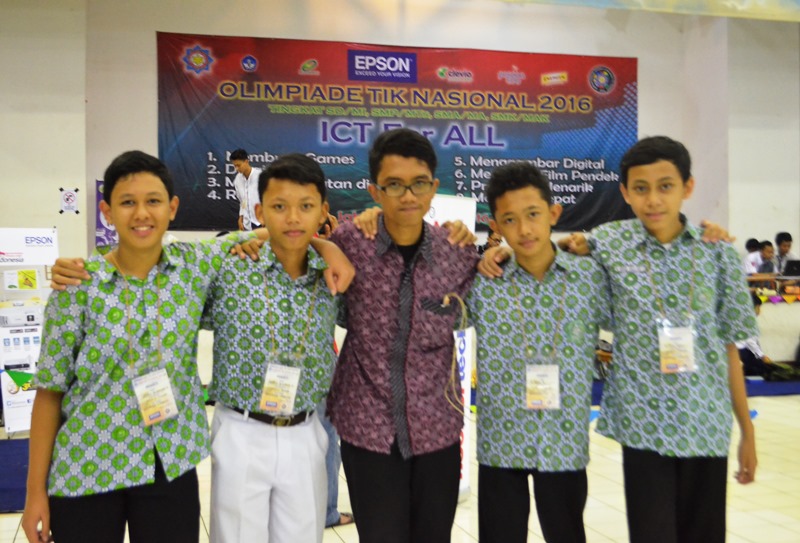This horizontal rectangular image, likely taken at a school fair, features five young men positioned in the center. The central figure, who appears to be an older individual possibly a teacher, is distinguished by his dark red shirt, black pants, and eyeglasses, with slightly longer black hair. Flanking him on either side are four school children, all seemingly of Indian descent and possibly aged between 8 to 12 years. Three of the boys wear matching dark green shirts adorned with white and green circles, while one boy at the far left wears a light green shirt with a similar pattern, differing slightly in shade. The boys sport black pants, except for one in white trousers, and all except the middle figure have name tags hanging around their necks.

In the background, a large banner prominently displays the word "Epson" at the top, followed by additional text and logos in a foreign language, possibly indicating sponsors for an event held in 2016. The banner has a gradient color scheme, transitioning from red at the top to brown, and then blue at the bottom. The background setting includes a white wall and other people sitting in the back right of the image. The group stands with their arms around each other, exuding a sense of camaraderie, with two of the boys smiling brightly.